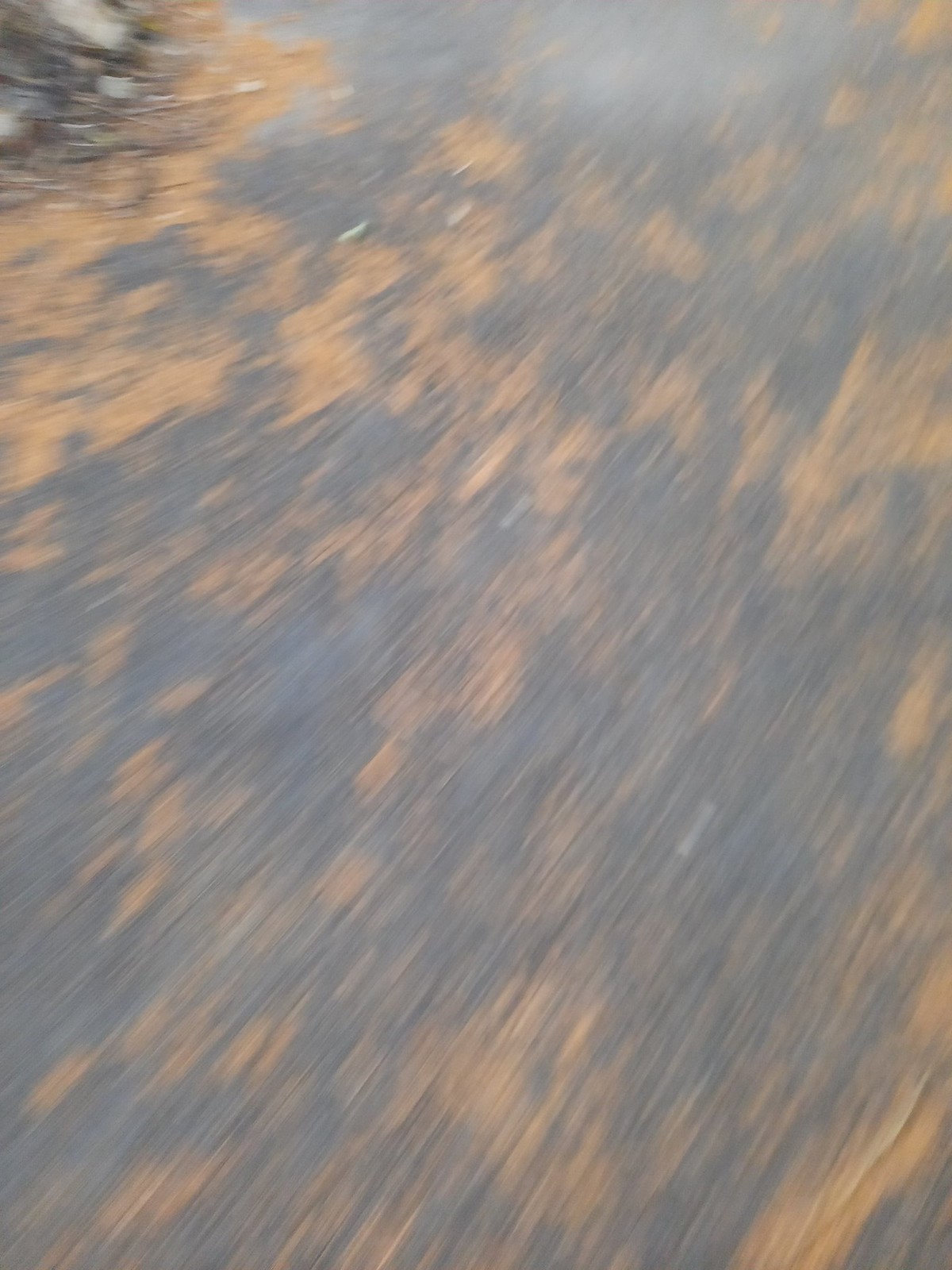The daytime outdoor photograph captures a blurry view of what appears to be a stone-covered walking path, littered with dried brown leaves. The image is dominated by motion blur, with streaks of gray and light brown running diagonally from the lower left to the upper right, making specific details difficult to discern. In the upper left corner, there is a slightly less blurred edge of the trail, which appears to have some rocks and twigs. Due to the motion blur, likely from the photographer moving while taking the shot, the scene is overall out of focus. The photograph is well-lit with natural light, emphasizing the dark and light brown hues of the ground and foliage.